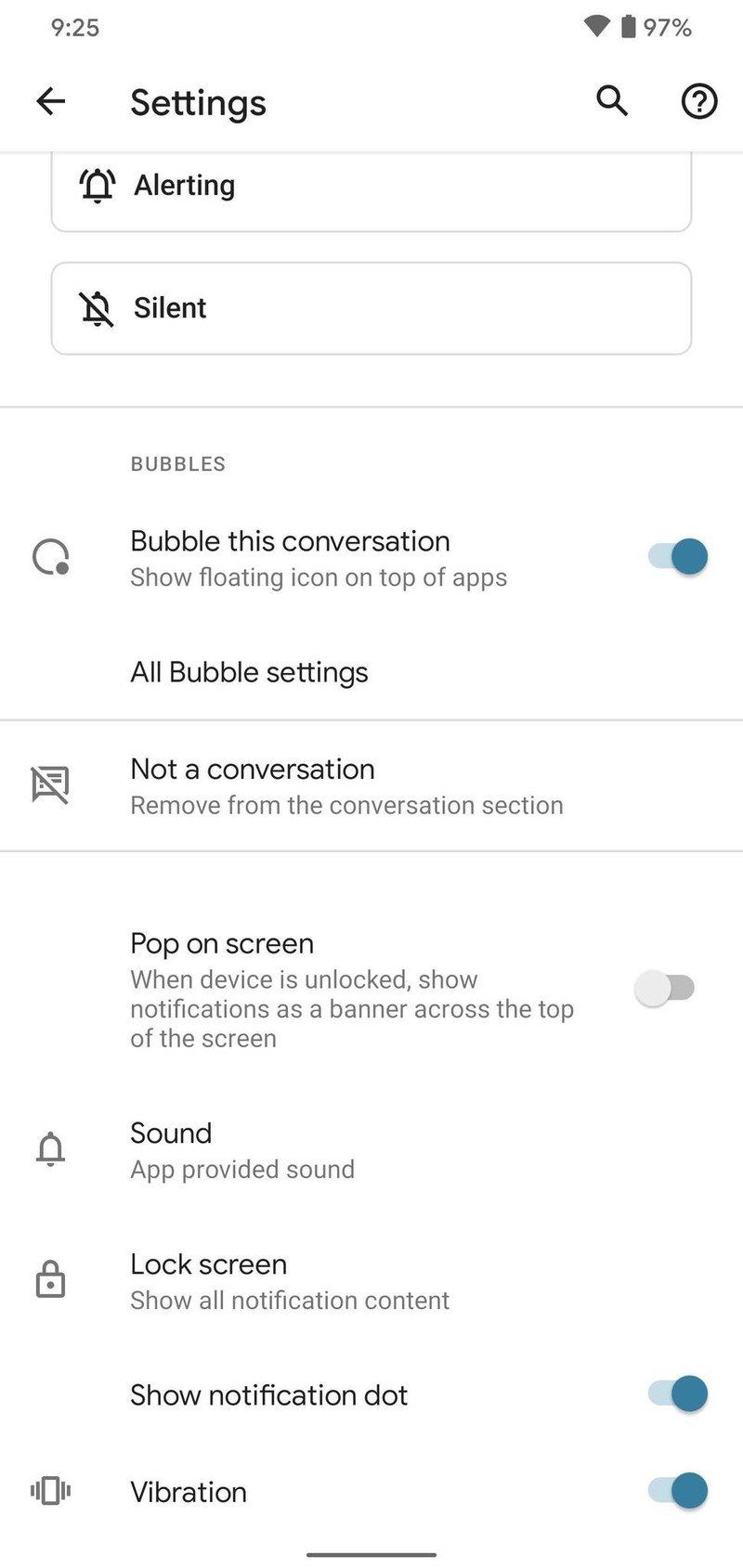### Descriptive Caption of the Screenshot:

At the top of the screenshot with a white background, the upper left-hand corner displays the time "9:25" in black text. The Wi-Fi signal icon next to the time is fully gray, indicating a strong connection, and the battery icon shows a 97% charge with the percentage displayed to its right.

Below these indicators, on the left-hand side, there is the word "Settings" starting with a capital "S." Next to it is a left-pointing arrow followed by a magnifying glass icon. Proceeding further to the right, there is a circled question mark icon outlined in black. A thin gray line separates this header from the subsequent content.

The next section features rectangular elements with light gray borders and black text. The words "ALERT" and "SILENT" are displayed prominently, separated by another thin gray line. Below, "BUBBLES" is written in all capital letters in gray, followed by "Bubble this conversation" in black. Underneath this, "SHOW FLOATING ICON ON THE TOP OF APPS" is written in gray.

Further down, the section header "BUBBLE SETTINGS" is in black, followed by a thin line. Then, "NOT A CONVERSATION" is written in black, with the instruction "REMOVE FROM THE CONVERSATION SECTION" in gray beneath it. 

After another thin line, the next black text reads "POP ON SCREEN," with the description "WHEN DEVICE IS UNLOCKED, SHOW NOTIFICATIONS AS A BANNER ACROSS THE TOP OF THE SCREEN" in gray.

Continuing downward, there is the word "SOUND" in black, followed by "APP PROVIDED SOUND" in gray beneath it. This pattern is followed by "LOCK SCREEN" in black, with "SHOW ALL NOTIFICATION CONTENT" written below in gray. Subsequently, "SHOW NOTIFICATION DOT" is listed in black, and at the very bottom, "VIBRATION" is written in black as well.